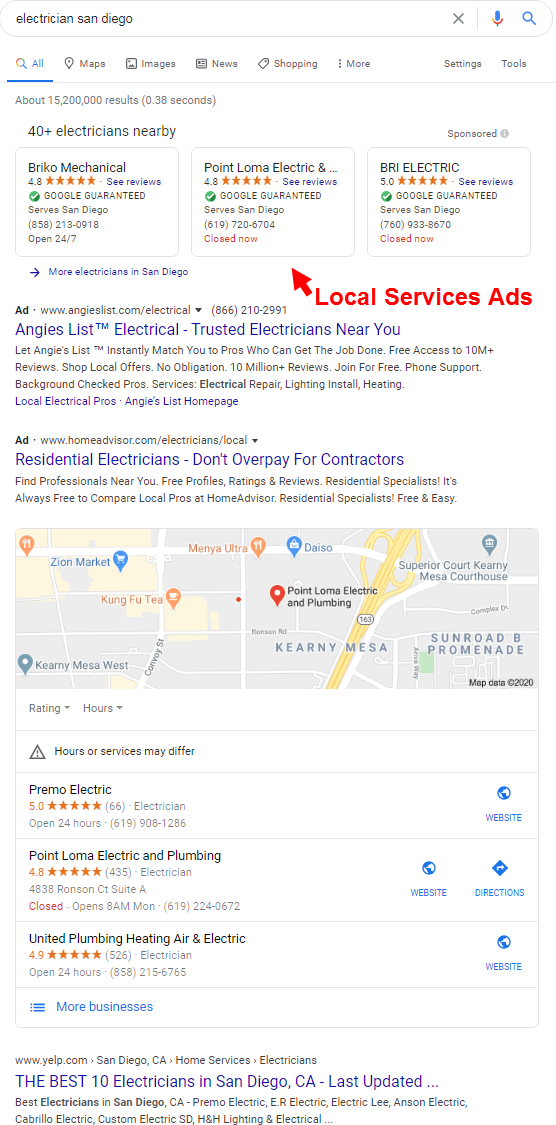In the image, we see a detailed Google search results page. The background is predominantly white with black text, interspersed with blue highlighted text and some orange icons. A prominent red arrow points to a specific icon, drawing attention to it.

At the top of the page, the search query "Electricians in San Diego" is visible within the search box. The "All" section is highlighted, with other options like Maps, Images, News, Shopping, and more settings/tools available but not selected. The search has yielded approximately 15,200,000 results.

Below the search bar, there are three highlighted boxes displaying information about local services. The results include "Berco Mechanical," "Point Loma Electrical," and "Bree Electric." Notably, "Point Loma Electrical" is underlined with a red arrow indicating a "Local Service Ads" feature, clearly pointing out its relevance.

Further down the page, the search results continue with listings such as Angie's List for trusted electricians near the user, residential electrician services, advice on avoiding overpaying for contractors, followed by a map section. Additional business results include "Primo Electric," "Point Loma Electric and Plumbing," "United Plumbing, Heating and Air Electric." Lastly, there's a section titled "Best 10 Electricians in San Diego, California," summarizing the top service providers in the area.